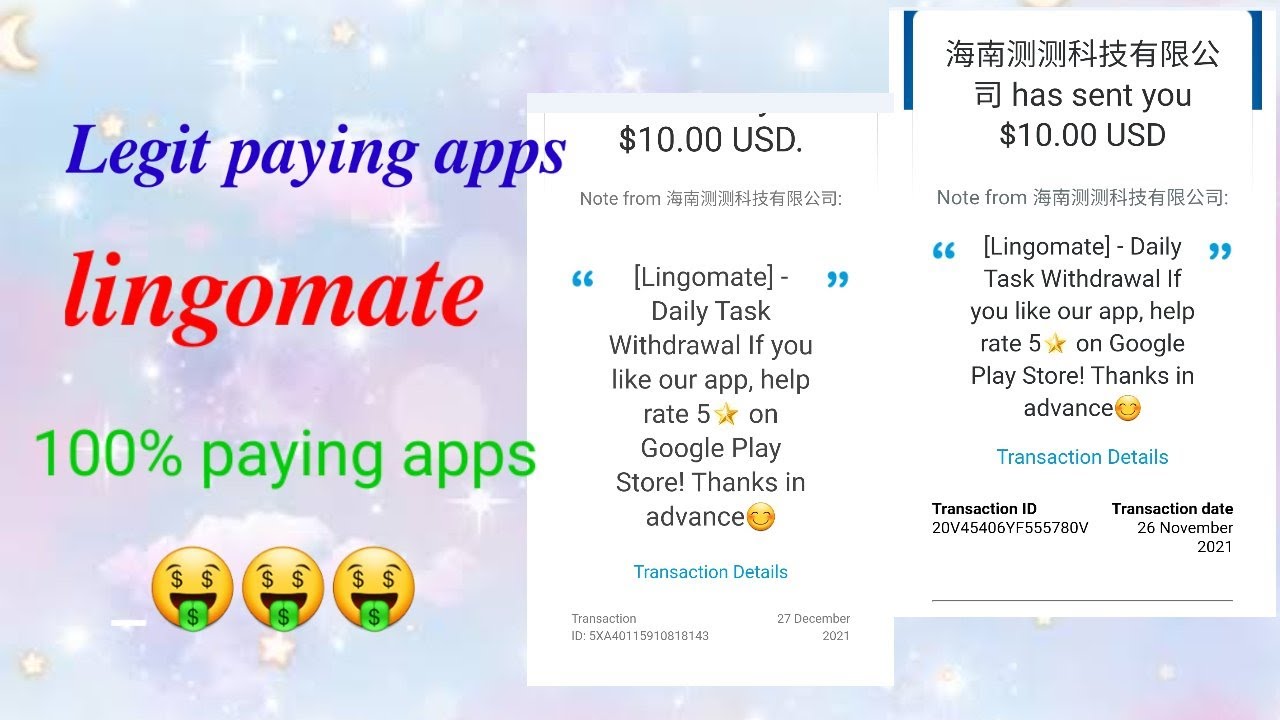**Advertisement for Lingomate:** 

This advertisement promotes "Lingomate," a platform for earning money through mobile apps. The website's background features a starry sky with clouds and a crescent moon in the top left corner. The headline, "Legit Paying Apps," is prominently displayed in blue letters. Below it, the app name "Lingomate" is highlighted in red, followed by the phrase "100% Paying Apps."

The advertisement includes three emojis of smiley faces with dollar signs for eyes and tongues sticking out, each holding green dollar bills. Adjacent to this section, there is a square indicating "$10 USD" followed by a message from a user profile in Chinese characters.

The message outlines: "Lingomate, daily task withdrawal. If you like our app, please rate us 5 stars on Google Play Store. Thanks in advance!" It also includes transaction details dated December 27, 2021.

Another identical message from the same user appears, confirming another $10 USD transaction dated November 26, 2021. Both messages emphasize withdrawing earnings through daily tasks and requesting users to rate the app five stars on Google Play Store. Each transaction is accompanied by a unique transaction ID.